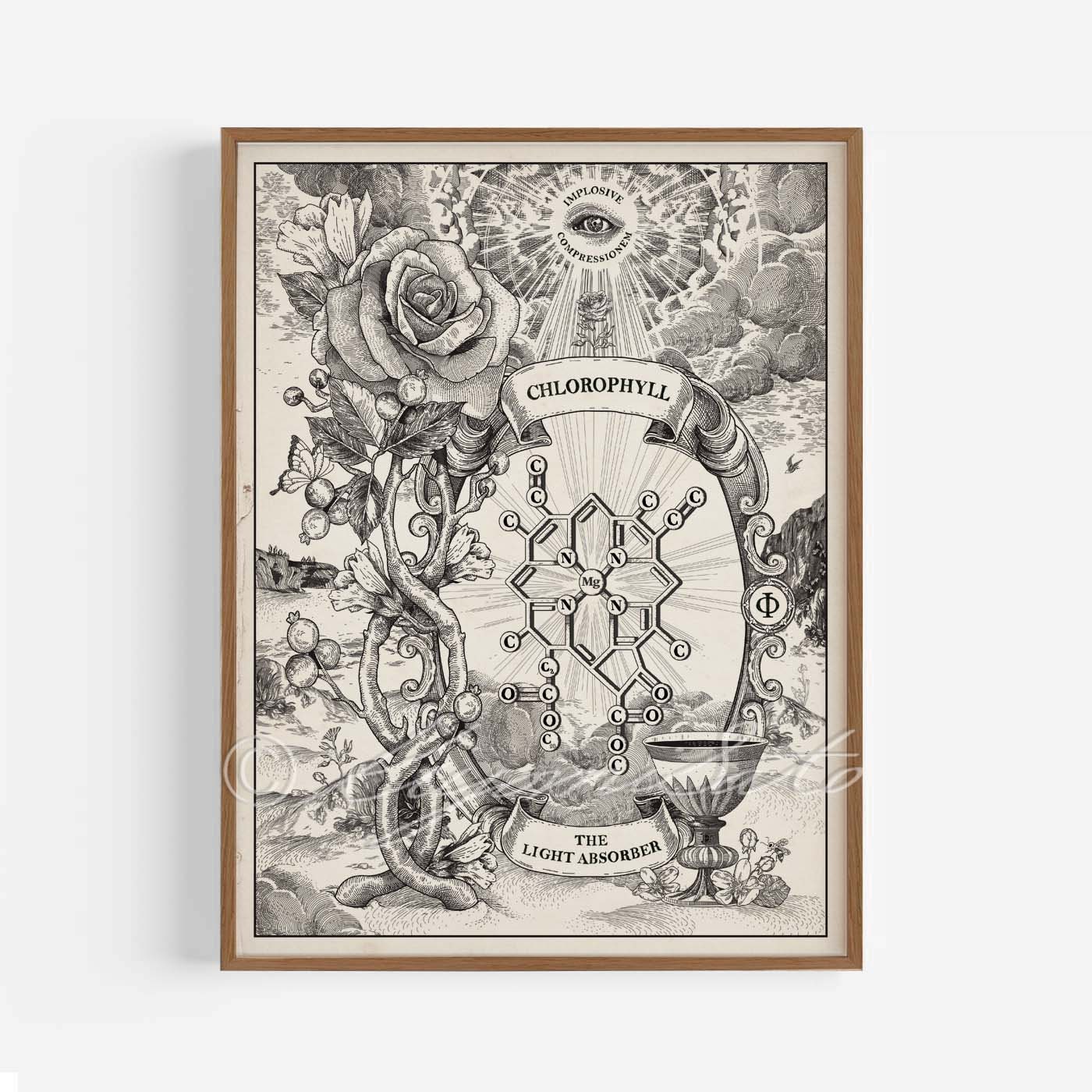This framed black and white drawing is a captivating and detailed artistic depiction of chlorophyll and its role in photosynthesis. The drawing is centered on a complex molecular structure, complete with chemical symbols representing elements such as carbon (C), manganese (Mn), oxygen (O), and nitrogen (N). Above this structure, the word "chlorophyll" is inscribed, while below it, the caption reads "the light absorber." 

At the top of the piece, the artwork features an eye symbolizing the sun, accompanied by the phrases "implosive compression" and "light rays," which are shown shining down through clouds onto a rose or flower, symbolizing the absorption of sunlight by plants. This intricate and thought-provoking piece hangs on a white wall, bordered by a small light brown wooden frame, making it both a scientific illustration and an evocative work of art.